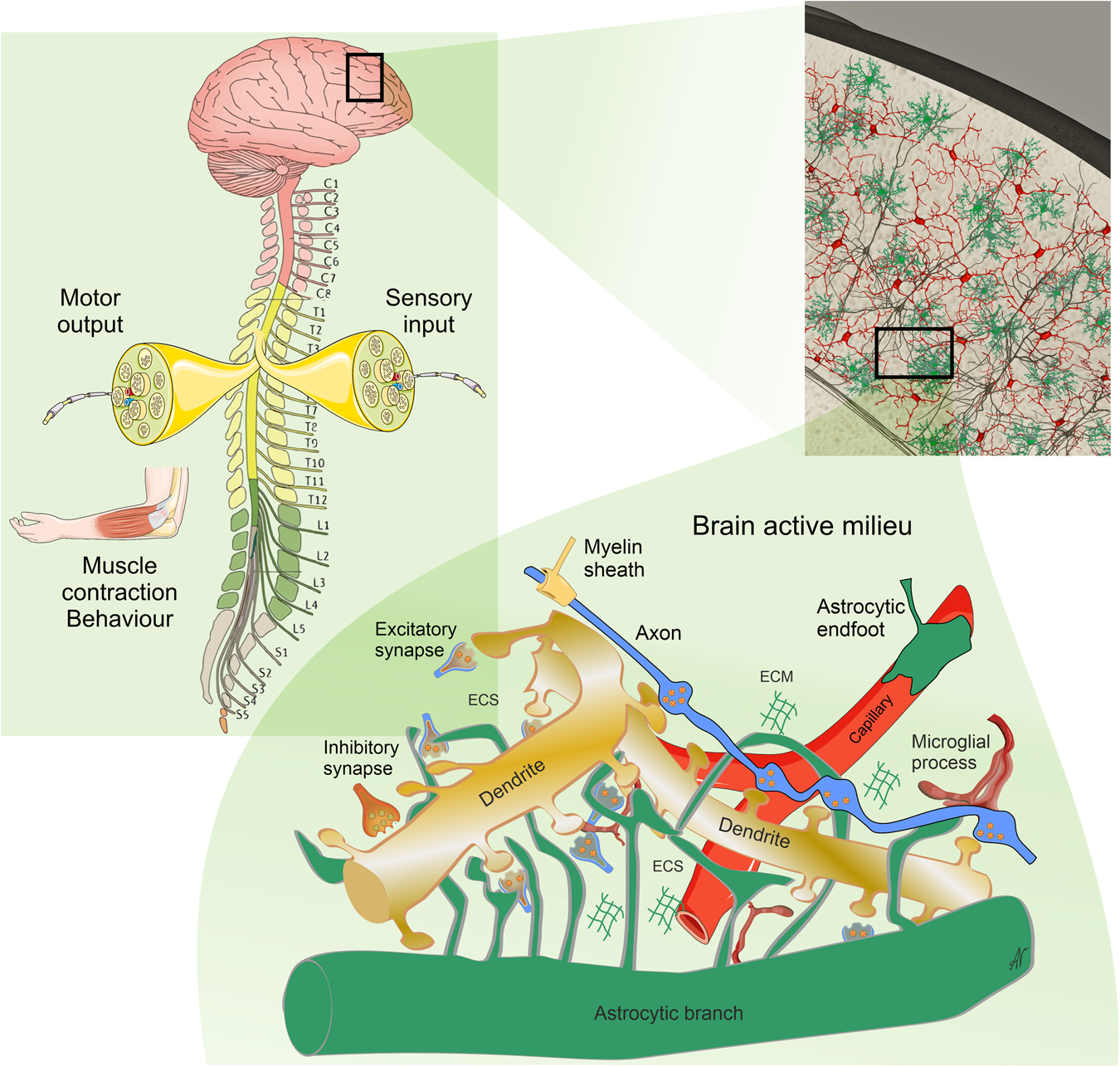This is a highly detailed, three-part medical diagram of human anatomy with a white background and highlighted sections in light gray showing the progression of magnification. The leftmost image features a comprehensive view of the central nervous system, depicting the brain connected to the spinal column. The spinal column is intricately labeled to indicate various vertebrae: cervical vertebrae (C1 to C8), thoracic vertebrae (T1 to T12), lumbar vertebrae (L1 to L5), sacral vertebrae (S1 to S5), and the coccyx. Additionally, it showcases a cutaway view of the spinal cord, illustrating motor output and sensory input pathways, along with an image of the forearm muscles labeled as "muscle contraction behavior."

In the upper right section, there is a close-up image of dendritic cells within the brain, displaying vivid green and red branching patterns against a white backdrop. This portion highlights the complex vascular structures in the brain.

Beneath this, in the lower right section, is an even more magnified view focusing on the intricate interactions within the brain. This detailed diagram showcases several dendrites, an astrocytic branch, a capillary, and multiple small synapses. This area is labeled "brain active milieu." The sequence of magnification moves from the overall view of the central nervous system to the dendritic cells and finally to the detailed synaptic interactions within the brain.